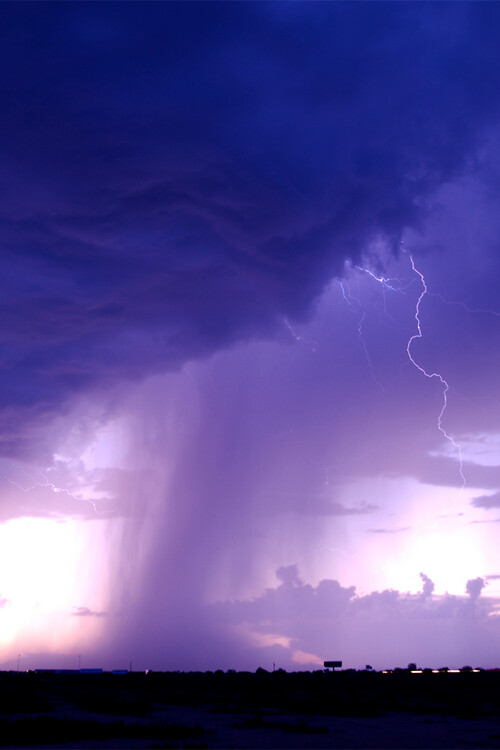The image depicts a dramatic vertical photograph taken during a severe storm. The sky showcases a breathtaking spectrum of purples, ranging from deep, dark purples to very light, almost whitish purple hues, highlighting the intensity and beauty of the storm. A prominent white lightning bolt can be seen striking down from the storm clouds, appearing to slice through the sky. The forefront of the image features dark silhouettes of what seems to be water, adding to the high contrast between the ominous stormy atmosphere above and the darker ground below. In the background, there are hints of distant buildings with lights on, partially obscured by the misty sheets of rain falling from the overcast clouds. The sky seems somewhat overcast with the storm cloud being extremely dark in the top left corner. The photo, triangular in shape, captures the raw power and beauty of nature in the midst of a severe storm, enhancing the drama with its monochromatic purple palette.